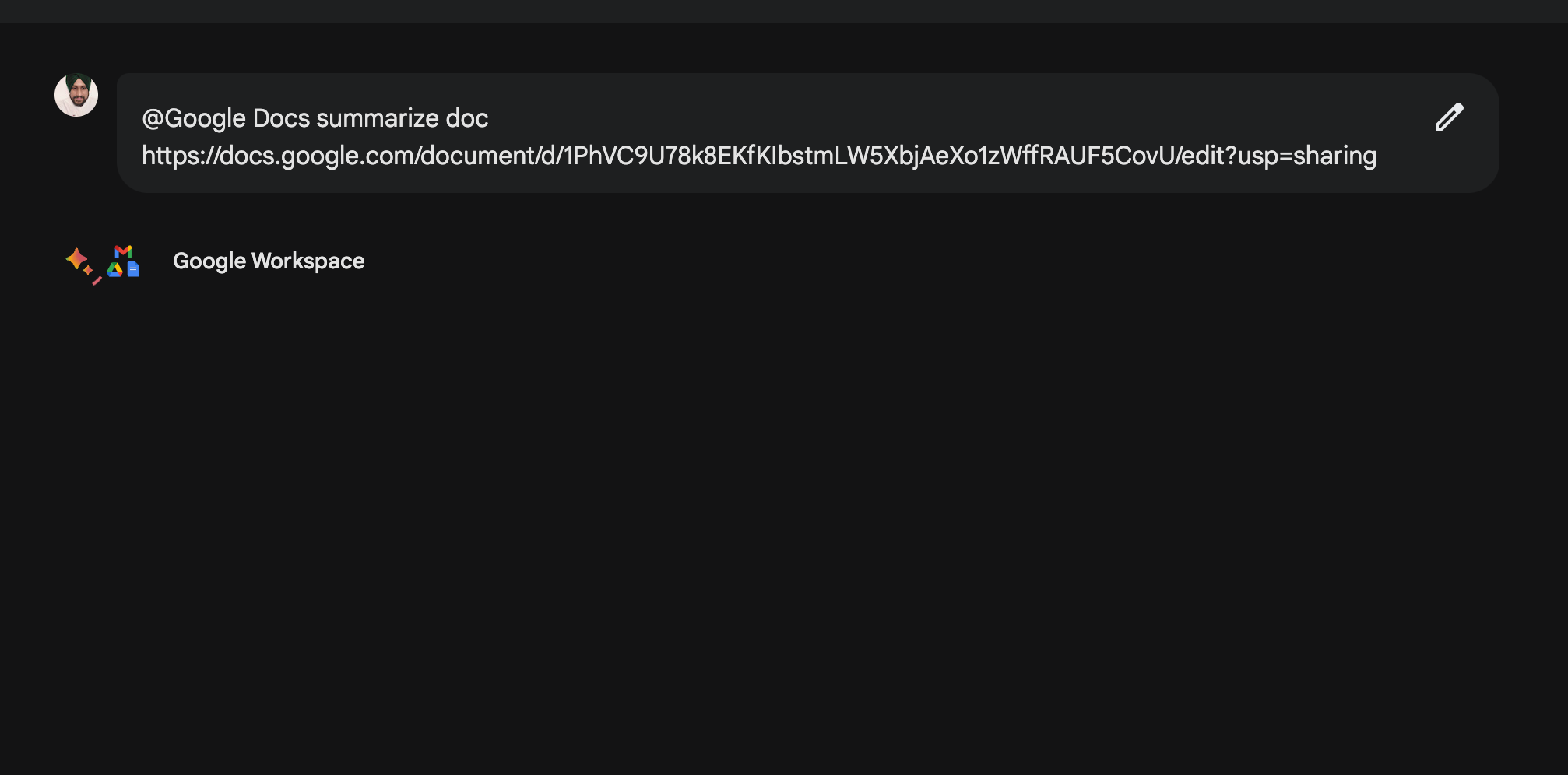This image is a landscape-oriented screenshot capturing a segment of a screen with a predominantly black background. At the very top, a thin, dark grey bar spans the entire width of the image. Just below this bar, in the upper left corner, there is a white circular icon containing a profile picture.

To the right of this profile icon, a long grey rectangle contains text in white font that reads, "Google Docs, summarize doc," followed by a link: "https://docs.google.com/document/d/1phvc9u78k8ekfklbstmlw5xbjaexo1zwffrauf5covu/edit? usp=sharing." In the top right corner of this grey rectangle, there is a simple white cartoon pencil symbol.

In the main section beneath, the words "Google Workspace" appear in large white text. To the left of this text, there are various smaller Google icons representing mail, share, and documents. These icons are significantly smaller in size compared to the elements above them.